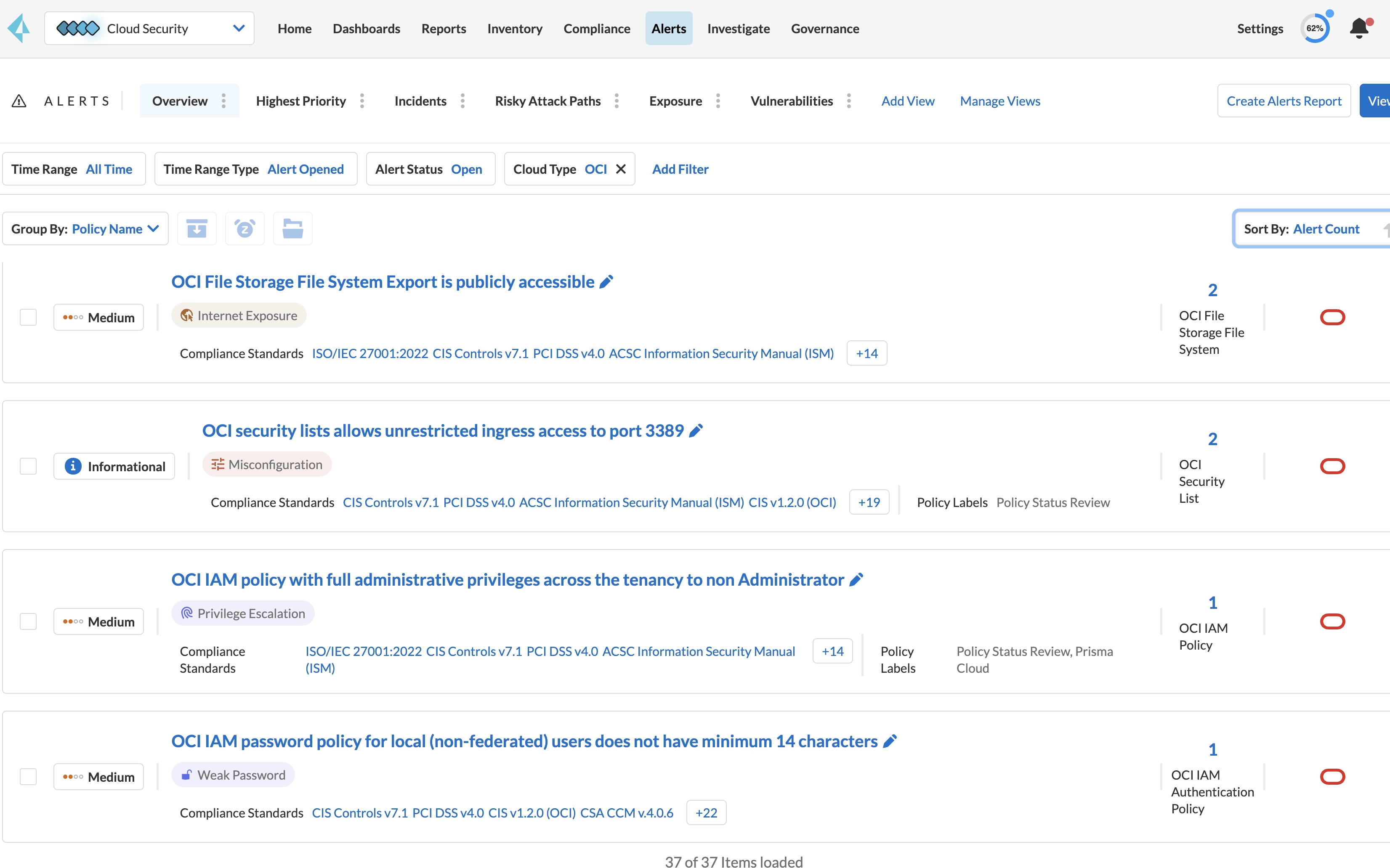This image is a screenshot from a cloud security company’s website. At the top, there is an icon comprised of four blue squares arranged like diamonds. To the right of the icon, the text "Cloud Security" is displayed, alongside a drop-down arrow.

Below this, a navigation menu features several clickable links, including Home, Dashboard, Reports, Inventory, Compliance, Alerts, Investigating, and Governance. The "Alerts" section has been highlighted, indicating it is the active page.

Within the "Alerts" section, the "Overview" tab is selected. The overview contains detailed information about various high-priority incidents and vulnerabilities. An itemized list of four alerts is displayed:

1. **OCI File Storage**:
   - Description: File system export is publicly accessible.
   - Issues: Internet exposure, compliance standards, etc.

2. **OCI Security List**:
   - Description: Allows unregistered ingress access to port 3389.

3. **OCI IAM Policy**:
   - Description: Provides full administrative privileges across the tenancy to non-administrators.

4. **OCI IAM Password Policy**:
   - Description: Does not require a minimum of 14 characters for local non-federated users.

Additionally, there is a lot of other text on the page that further details these alerts and their implications for cloud security.